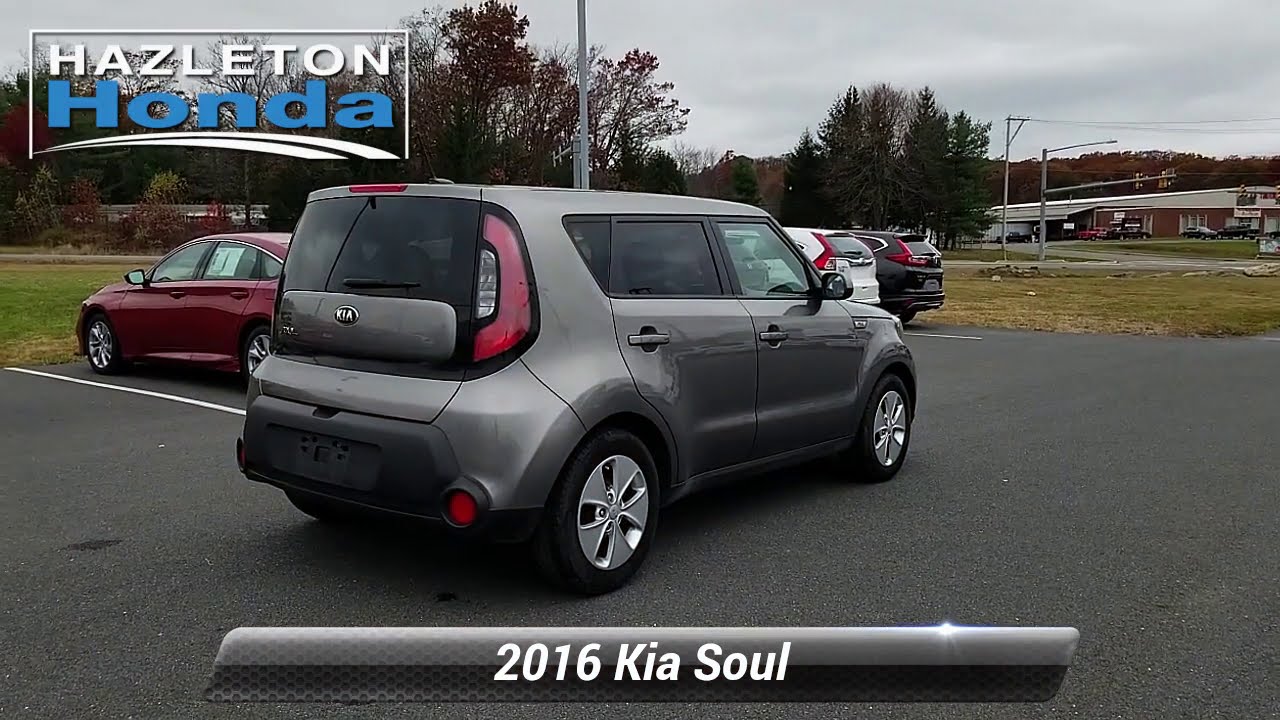This image features an advertisement for a 2016 Kia Soul from Hazleton Honda. Positioned in the center on dark gray pavement, the gray, somewhat boxy Kia Soul is facing away from the camera at a diagonal angle, revealing its red taillights, tinted windows, and silver wheels. The rear of the car prominently displays the Kia logo. Superimposed on the top left corner of the image is the dealer's logo, "Hazleton" in white and "Honda" in blue with a white swoosh beneath. At the bottom of the image, in a shiny black rectangle, reads "2016 Kia Soul" in white text. The parking lot surrounds the car, showing several other vehicles, including a red car and a white and black SUV. The background features a grassy area, a forest with predominantly dark trees, and a commercial building in the top right corner. The overall setting is during an overcast daytime, indicated by the gray cloudy sky above.